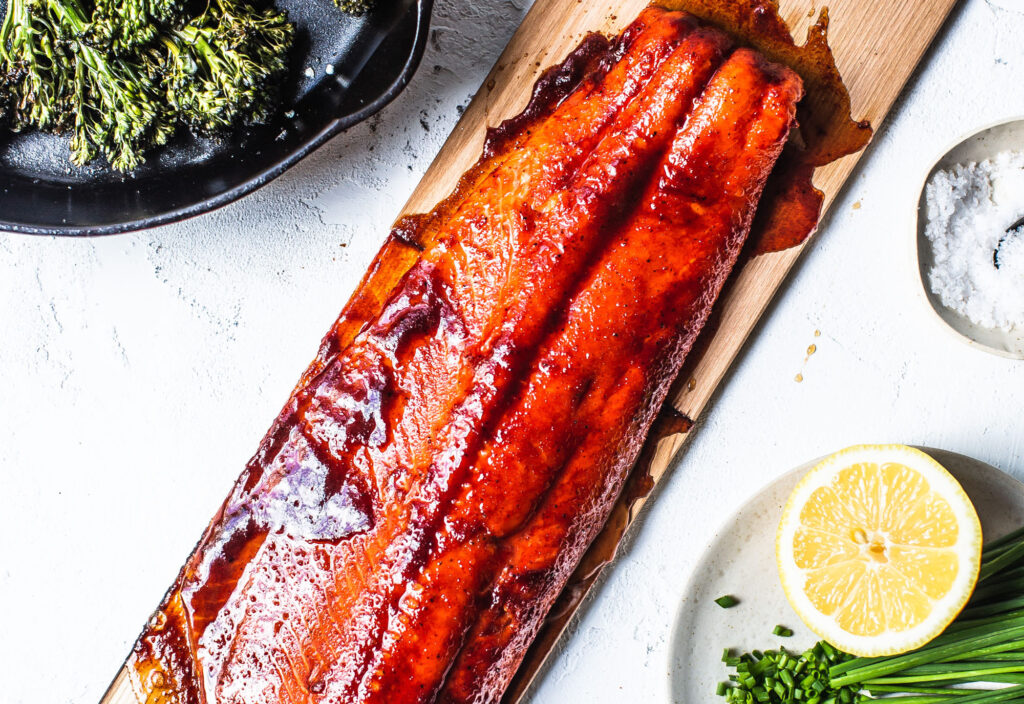This photo presents an overhead view of a professionally photographed and vibrant barbecued fish dish, likely salmon due to its texture, layered with a rich red sauce. The fish rests on a thin wooden cutting board atop a white counter. Just above to the left, a black skillet contains either asparagus or broccolini, suggesting it was cooked or fried. To the right of the wooden board, a ceramic off-white plate holds a yellow lemon half, showcasing visible flesh. Additionally, the scene includes some chopped scallions on the plate, beside which lies a small bowl of white salt. The displayed arrangement and meticulous preparation imply this image was created for a food blog or an Instagram post.